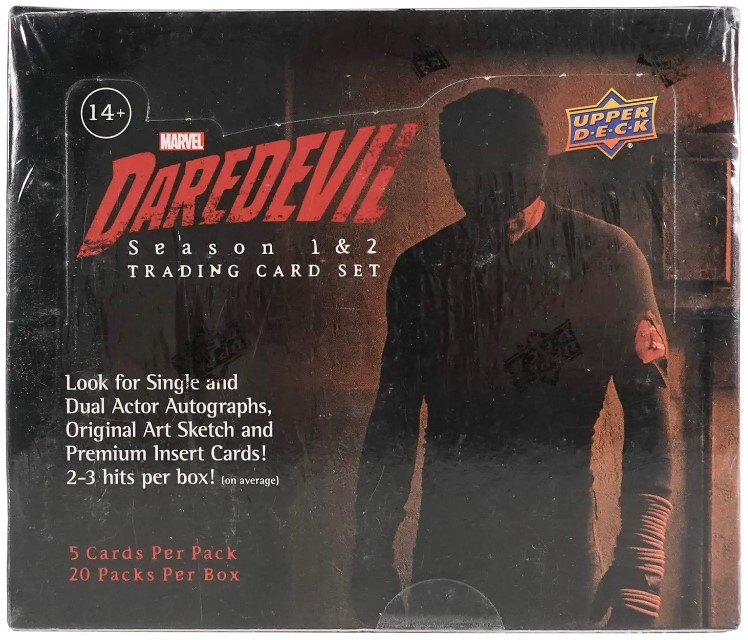This image features a dark, atmospheric advertisement for the Marvel character Daredevil, specifically highlighting the Daredevil Season 1 & 2 Trading Card Set by Upper Deck. The ad shows a masked Daredevil looking down, cloaked in a long-sleeve shirt and black gloves. Prominently, the Upper Deck logo appears in yellow and blue on the top-right, while the Marvel logo in its iconic red and white is positioned to the left with a circle indicating "14+" just above it. Below the Marvel logo, "Daredevil" is boldly written in red uppercase letters in a unique font, followed by "Season 1 & 2 Trading Card Set" in white. 

The advertisement entices collectors with promises of potential finds, stating: "Look for single and dual actor autographs, original art sketch, and premium insert cards. 2-3 hits per box (on average)." Further details note that each box contains 20 packs, with 5 cards per pack. The top of the box, scanned in the image, still shows its plastic wrapping and tape, preserving its unopened, collectible state. There is also a push-down tab designed to open the box.